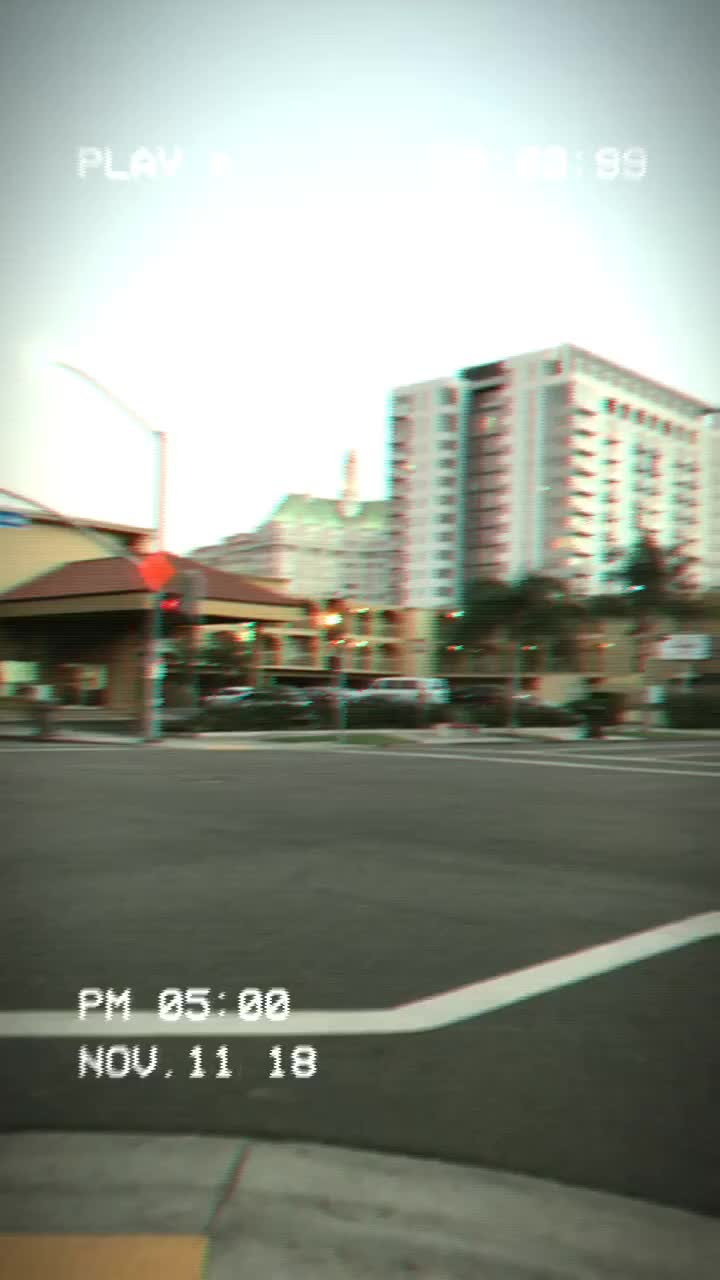The image appears to be a low-resolution, surveillance camera shot from a street corner, timestamped "PM 05:00, November 11th, 2018." The scene captures a cityscape under an overcast sky. A streetlight can be seen on the left, and white street markings are visible on the asphalt. There are also concrete curbs bordering the street. In the background, there are several buildings, including a large white hotel with some brown detailing and a smaller building that could possibly be a bank drive-through due to its distinctive roof structure. The scene includes some parked cars and palm trees, adding to the urban atmosphere. An orange, four-pointed, triangular sign is also visible, indicating some form of notice or warning.